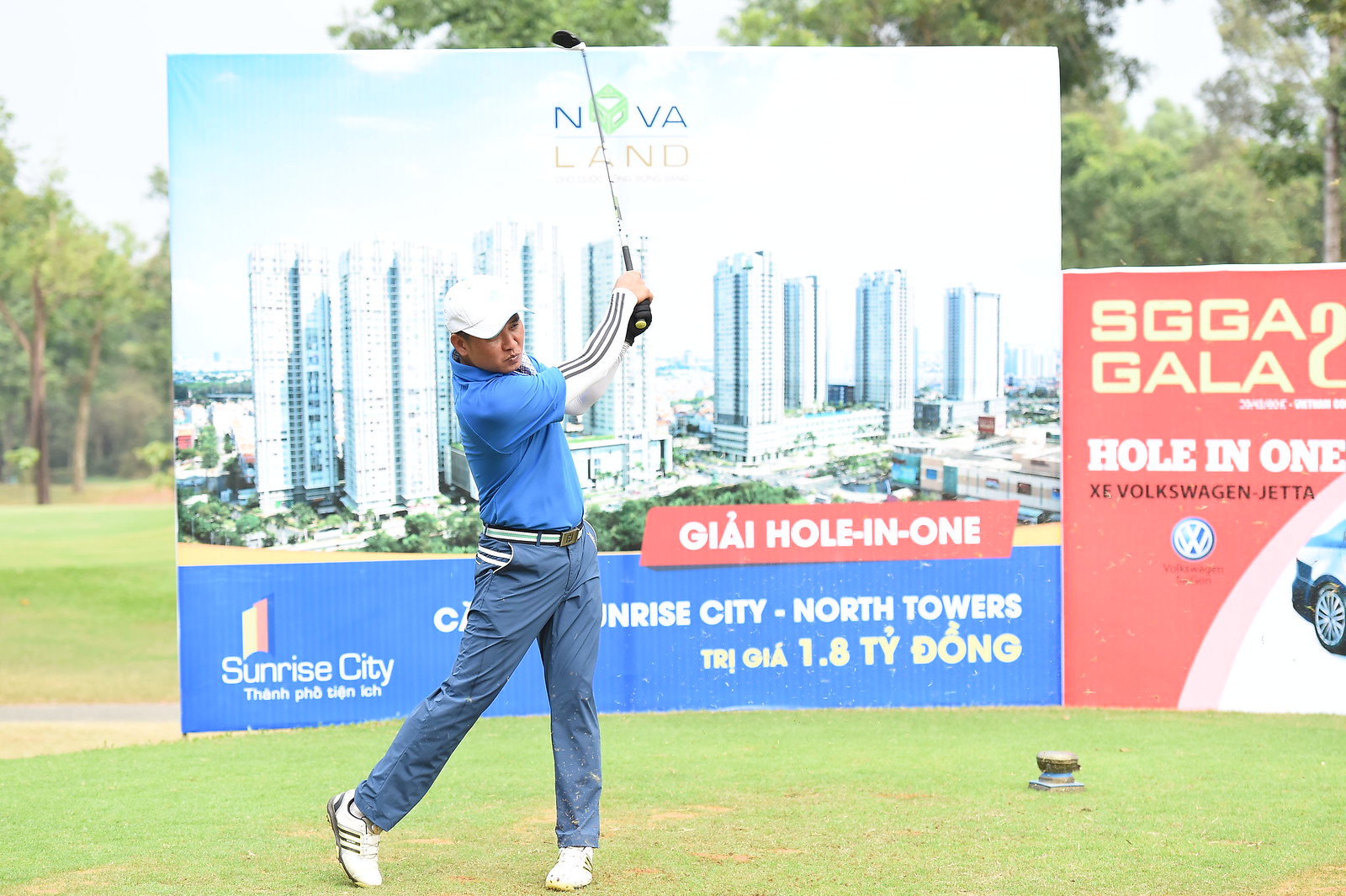In the image, an Asian golfer is captured mid-swing on a grass tee, set against a backdrop of large advertisement signs with an array of text and images. He is wearing a blue short-sleeved polo shirt layered over a white long-sleeved shirt with black stripes running down the arms, a white hat, light blue pants, a white belt, and white golf shoes with black stripes. 

The largest sign prominently features the word "NOVALAND" at the top, below which is an image of high-rise apartment buildings in a metropolitan setting. The text beneath this image reads "GIAI Hole-in-One" on a red background with white letters. Further down, it states "Sunrise City North Towers" with "Sunrise City" in white on a blue section at the bottom.

Adjacent to this sign, to the right, is a red sign with partially visible text: "SGGA" at the top, followed by "GALA" and "Hole-in-One XE Volkswagen Jetta," along with the Volkswagen logo below it.

The surrounding area is lush with trees, and the golfer's mid-swing pose suggests he is participating in a golfing event, possibly sponsored by Volkswagen Jetta, as indicated by the signage.